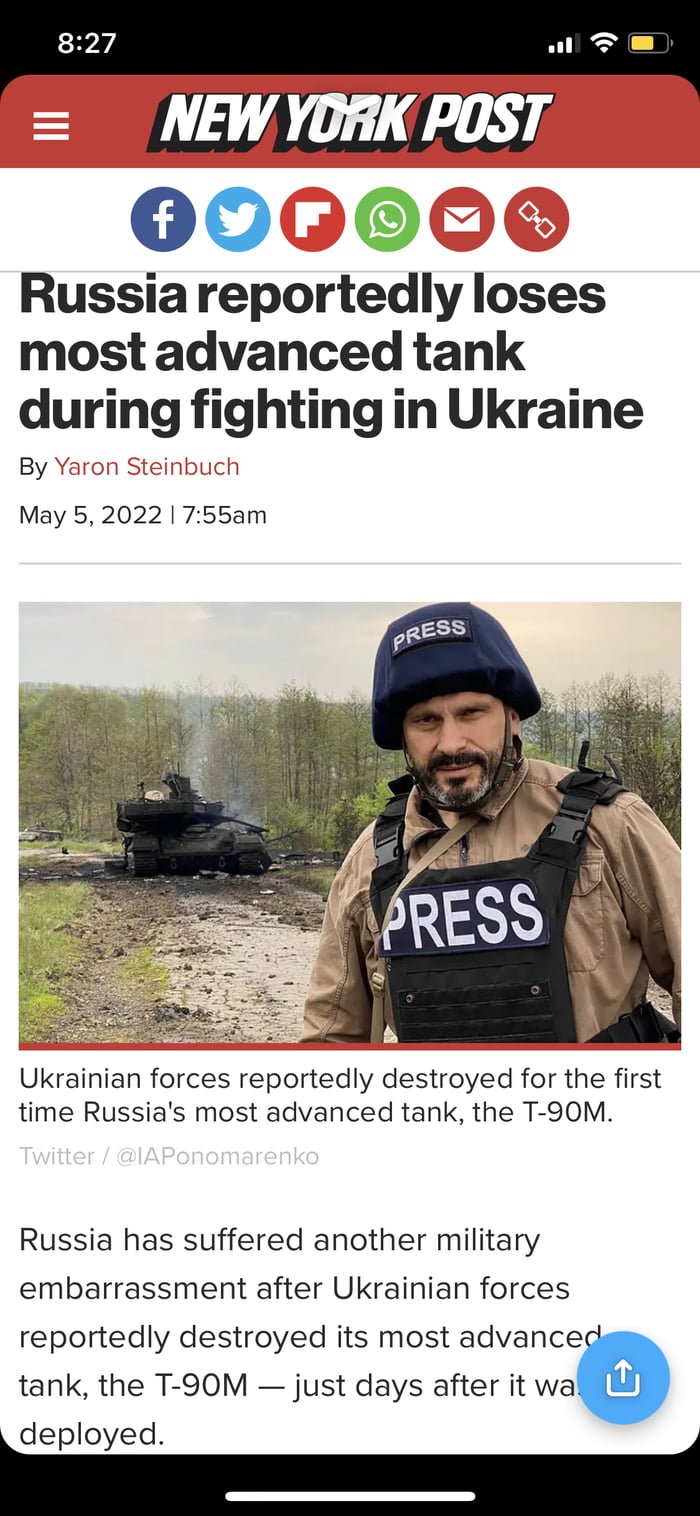**Caption:**

A screenshot of a New York Post article is captured on a smartphone screen. At the top of the screen, the black header of the phone shows the time as 8:27 AM on the left, and on the right, it displays the phone's status icons – a 4G signal with three vertical bars, a Wi-Fi symbol indicating full connectivity, and a yellow battery icon showing approximately 65% charge.

Below the phone's header, the New York Post logo is prominently displayed with a red three-bar menu icon to its left. Directly beneath this is a white strip containing several social media and sharing icons – Facebook, Twitter, an unidentified icon, WhatsApp, email, and a chain link for sharing.

The article's headline, "Russia Report Loses Most of the Land's Tent During the Fighting in Ukraine," is boldly printed beneath the icons. The byline attributes the article to Yaron Steinbuch, dated May 5th, 2022, with a publication time listed as 7:55 AM to the right of the date.

The article is accompanied by an image of a bearded man wearing a press uniform, positioned behind what appears to be a tank. The image has a blueish tint, and additional text related to the article and a share or download button can be seen below the picture. A black bar spans the bottom of the smartphone screen, completing the display.